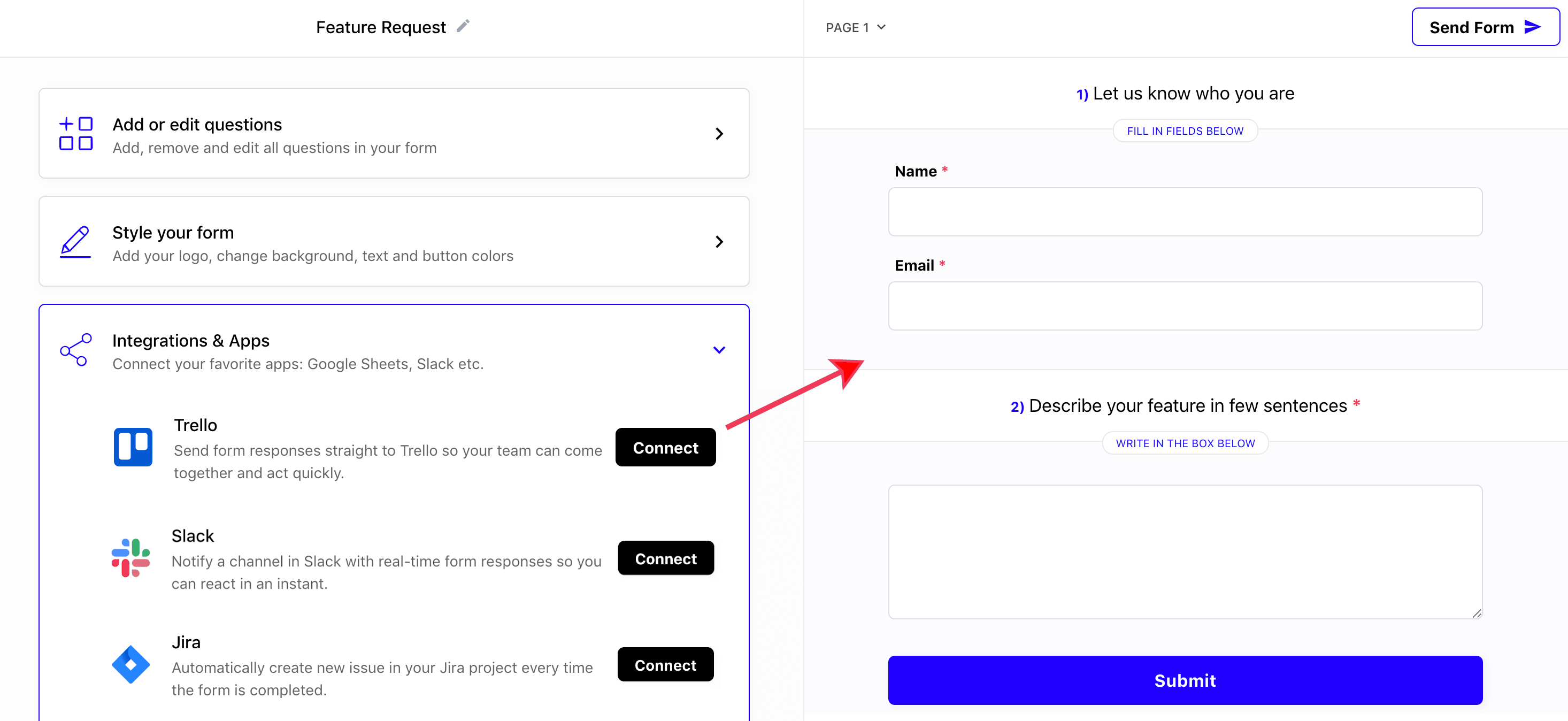In this image, there is a page displaying future requests. A pencil icon, symbolizing the option to edit, is located to the right of each future request. Various options for customization and integration are outlined on this page. Users can add or edit questions, remove or modify all questions within their form, and personalize the form's appearance by adding a logo or changing the background, text, and button colors. Integration options include connecting with favorite apps such as Google Sheets, Slack, and Trello. For example, users can send form requests directly to Trello to facilitate team collaboration. Integration with Slack allows real-time form responses to notify specified channels for prompt reactions. Additionally, completing the form can automatically create new issues in a Jira project, streamlining project management.